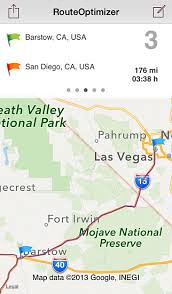This screenshot, taken on a phone, showcases a route optimization application. At the top of the screen, the app is titled "Route Optimizer." On the left side of the title bar, there is an icon depicting a square with an upward-pointing arrow, and on the right, a square icon that resembles a pencil, indicating editing functionality.

Below the title bar, there is a green flag marker labeled "Barstow, CA" for Barstow, California, USA, accompanied by a large number "3" to its right. Beneath this, an orange flag marker indicates "San Diego, CA, USA," noting a distance of 176 miles and an estimated travel time of 3 hours and 38 minutes.

Further down, there are five dots with the middle dot highlighted, possibly indicating the current view or step in the route. The subsequent large section displays a map with various names and small map graphics. In the top left corner, partially obscured text reads "Death Valley National Park," missing the initial 'D' and 'NA' due to cropping. To the right, "Las Vegas" is labeled with a blue flag next to it.

Above and slightly to the left of Las Vegas, the town of "Pahrump" is marked. The optimized route is displayed in a highlighted path, beginning in Las Vegas and stretching southwest to "Barstow," which also bears a blue flag. The route passes through the Mojave National Preserve and near the town of Fort Irwin. At the bottom of the map, there is a notation: "Map data ©2013 Google, INEGI."

This screen effectively illustrates a planned journey through several notable locations, providing key visual and textual information regarding the route.